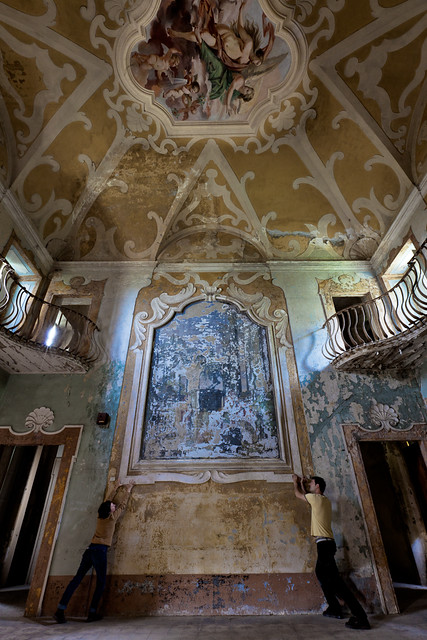This photograph depicts the interior of a grand, possibly hexagonal or pentagonal, two-story room reminiscent of a 17th-century church, marked by its various shades and states of stone disrepair. The main feature on the bottom floor is a large, inlaid painting on a distressed main wall, framed by two large doorways. Two people, a man in a yellow shirt and black pants, and a woman in a brown shirt and black pants, are seen adjusting the frame of this painting, which exhibits significant damage with chipped colors. Gold and muted blue tones dominate the artwork, which hints at biblical scenes yet is indistinct due to the wear. Above, the ceiling showcases a painted fresco with floral flourishes, centered around a panel, also likely depicting a biblical scene. The second story has balconies with scrolled metal railings leading off into doorways, suggesting exterior access based on the streaming light. The subtle interplay of gold, light pink, and cream hues on the ceiling and fresco add to the room’s regal, yet faded, splendor.